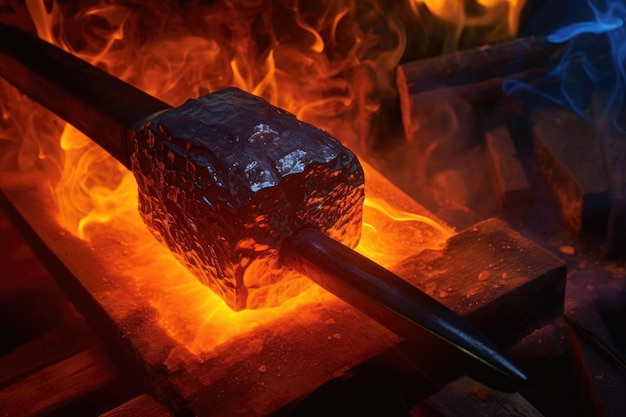The image appears to capture a vividly lit blacksmith's forge, featuring a prominent, dark, iron spike piercing through a roughly finished black stone, possibly onyx. The stone, shaped like an elongated cube with chipped edges reminiscent of ancient stonework, is positioned approximately six inches from the pointed tip of the spike, which descends diagonally from the upper left to the lower right. Beneath this setup, intense flames flicker, emitting a striking orange glow that merges with a surrounding blue light, creating a fantastical, almost surreal atmosphere. The detailed, high-resolution quality of the image, combined with the impeccable lighting of the scene, imparts a fantasy-like quality that raises questions about whether the image is a realistic photograph or a sophisticated computer-generated visual.